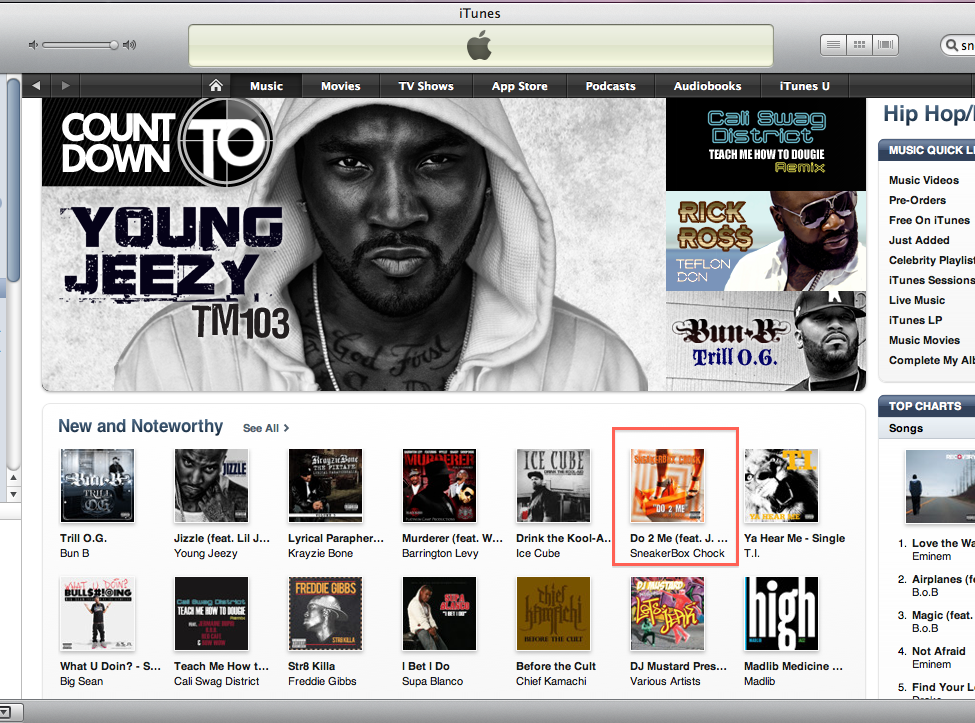This image is a horizontally-oriented screenshot of the iTunes web page. The interface is characterized by a silver address bar at the top, where "iTunes" is prominently displayed in the center. The address bar features an Apple icon and has a very light yellow hue. Just below the address bar, there is a categorized navigation list including "Music," "Movies," "TV Shows," "App Store," "Podcasts," "Audiobooks," and "iTunes U." The "Music" category is currently selected.

In the top-left corner of the main content area, there is a promotional banner titled "Countdown to Young Jeezy TM103." Accompanying the text is an image of an African-American man with a beard, dressed in a white hoodie, directly engaging the viewer with his gaze. To the right of this banner, the names "Cali Swag District," "Rick Ross," and "Bun B" are listed, indicating other featured music acts available for purchase.

Adjacent to this section is a selection box containing miscellaneous music-related options. In the lower right-hand quadrant, there is a "Top Charts" section, enumerating the most popular songs currently available.

At the bottom of the page runs a horizontal section labeled "New and Noteworthy." This section showcases fourteen different musical acts, distributed in two rows of seven. Each act is represented by an icon featuring the album cover above the name of the artist or band.